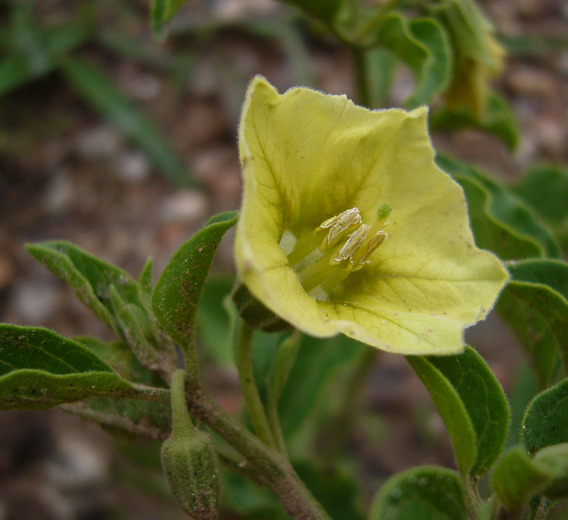This close-up, square photograph captures a vivid outdoor scene featuring a prominent yellow flower, likely resembling a tulip, as its central focus. The flower, displaying jagged yellow petals with green veins and subtle white edges, stands out sharply against a richly blurred background. The petals curve gently, enveloping a central structure with light yellow pollen and a lime green-tipped stigma, all of which are intricately detailed and in clear focus. The surrounding plant includes numerous green leaves, which are pointed, curled, and reminiscent of cups that might hold rainwater. These leaves are part of the same plant and add a lush contrast to the overall composition. The background is a blend of rich brown soil, suggestive of mulch or autumn leaves, interspersed with white spots resembling stones. The blurred backdrop further includes hints of additional greenery and rustling leaves, enhancing the natural and serene wooded setting of this image. The colors present—yellow, green, brown, white, and black—complement each other, providing a detailed and harmonious representation of this vibrant slice of nature.